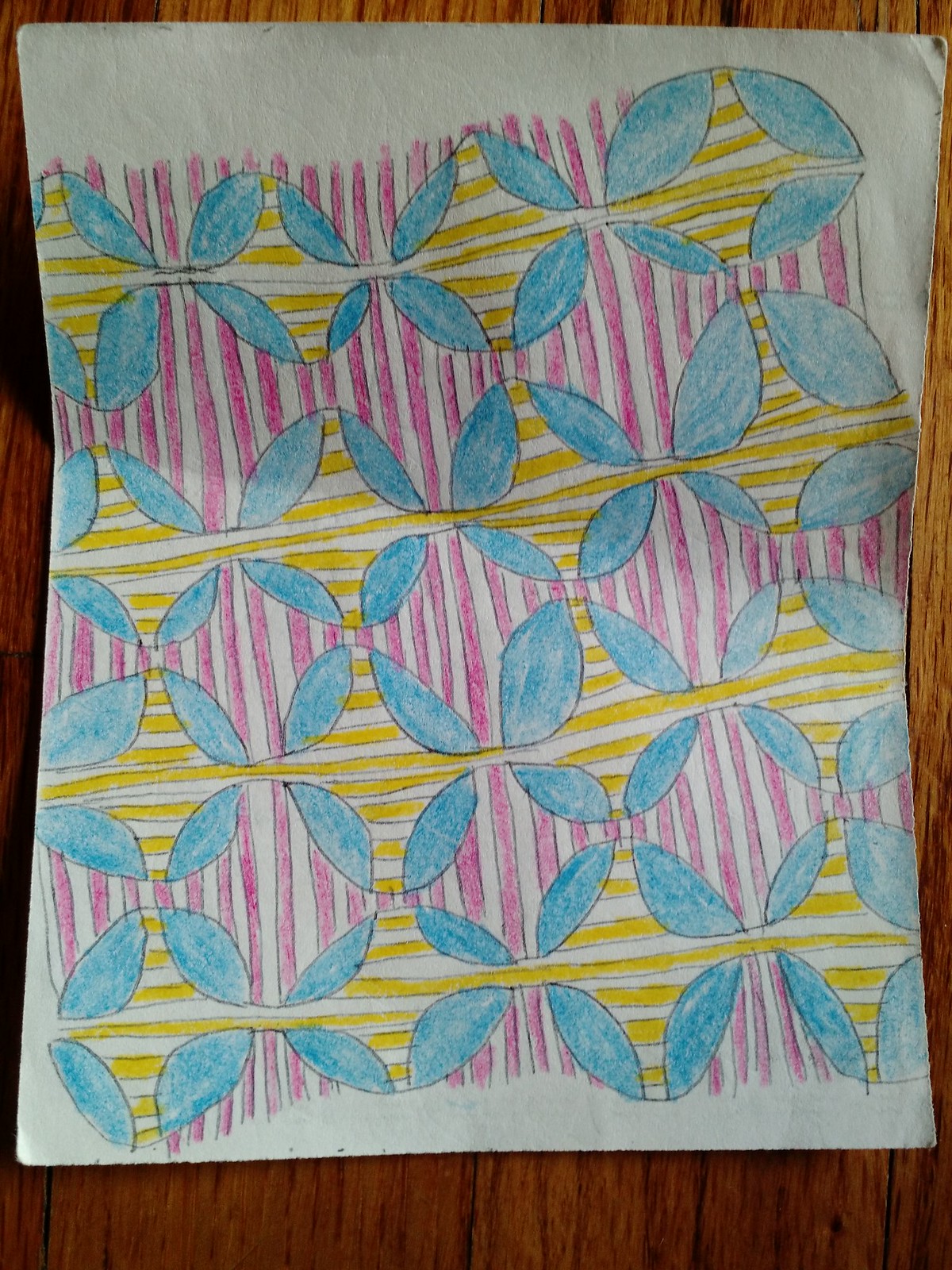The image is a detailed drawing on a white sheet of paper, which is placed on a brown table. The paper has slight wrinkles in the top right corner and ruffled edges along the right side. The artwork features a complex woven pattern composed of pink and yellow lines. There are six vertical pink stripes and yellow stripes running horizontally across the design. Interspersed within this grid are blue flower-like circles, totaling four evenly spaced flowers. Two circles are positioned at the top and two at the bottom, with their petals pointing in the cardinal directions (northeast, southeast, northwest, and southwest). The blue flowers have their petals delicately shaded in a light blue color. The top left corner of the paper remains uncolored, while the rest is meticulously filled in, giving it an appearance reminiscent of a quilt.